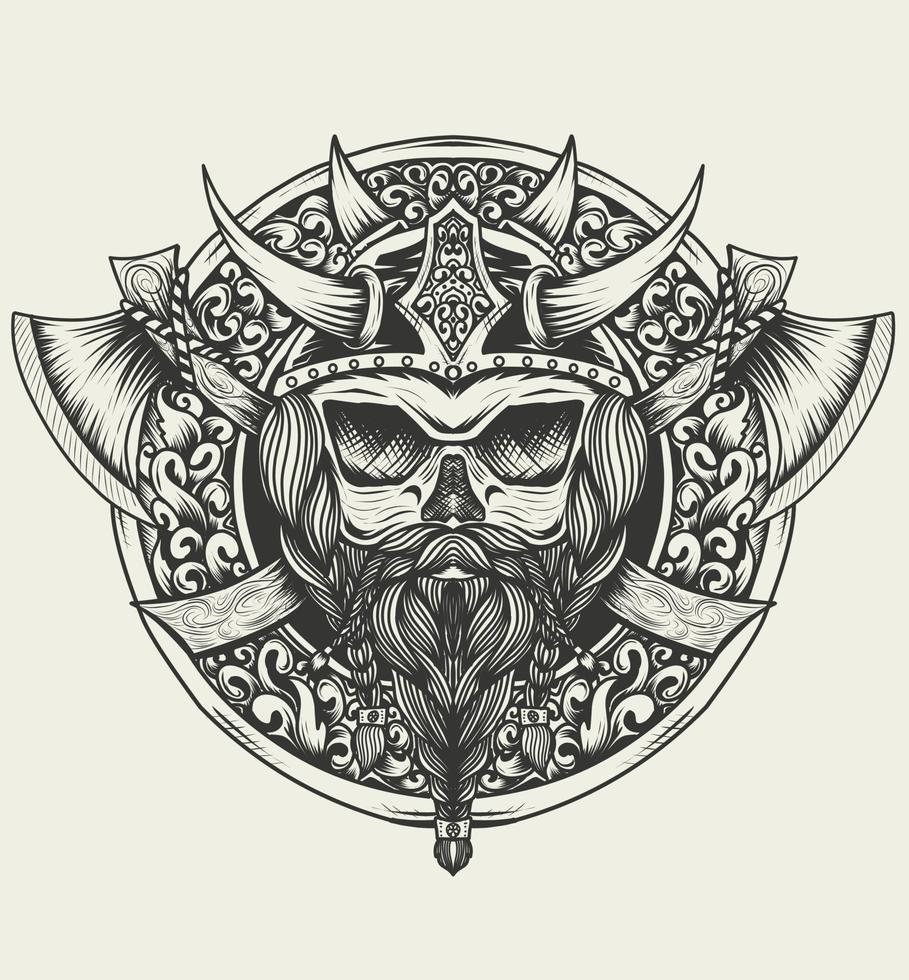This digital artwork, rendered entirely in black and white with an off-white, tannish background, depicts a striking Viking-themed emblem or potential tattoo design. Central to the image is a menacing Viking skull with hollow eyes and a dark, hollow nose, giving it a somewhat skeletal appearance. The Viking wears a horned helmet, with four protruding horns—two at the front and two at the back—and intricate, ornate decorations. The Viking’s facial features are meticulously detailed; it sports a long, braided mustache and a beard adorned with a small jewel at the end. Long, braided hair frames each side of the skull. Crisscrossing behind the Viking head are two wide-bladed axes, with visible twine bindings adding to the rustic aesthetic. The entire composition is enclosed in a round emblem, embellished with intricate, flowing filigree patterns, reminiscent of medieval designs. The highly detailed artwork, characterized by its stylized line drawings and shading, suggests its suitability as a tattoo, game logo, or similar emblematic representation.